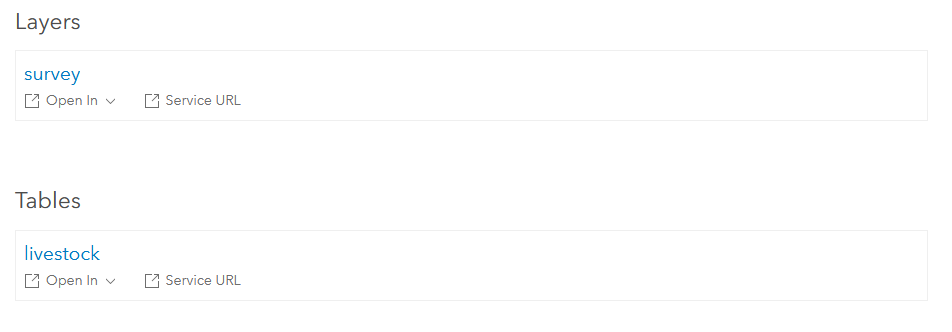The image showcases a minimalistic user interface or webpage layout against a stark white background. Dominating the upper section of the page are two prominent rectangular boxes. The first box, labeled "Layers," is positioned at the very top of the page. Directly beneath this box, there is the word "Survey," accompanied by an "Opt-In" button and a "Service URL" button. The second rectangular box, titled "Tables," contains sub-sections or options listing items such as "Livestock," "Open In," and "Service URL." The overall design is extremely straightforward and uncluttered, focusing solely on these two boxes without any additional elements, graphics, or text, emphasizing its basic and simplistic aesthetic.